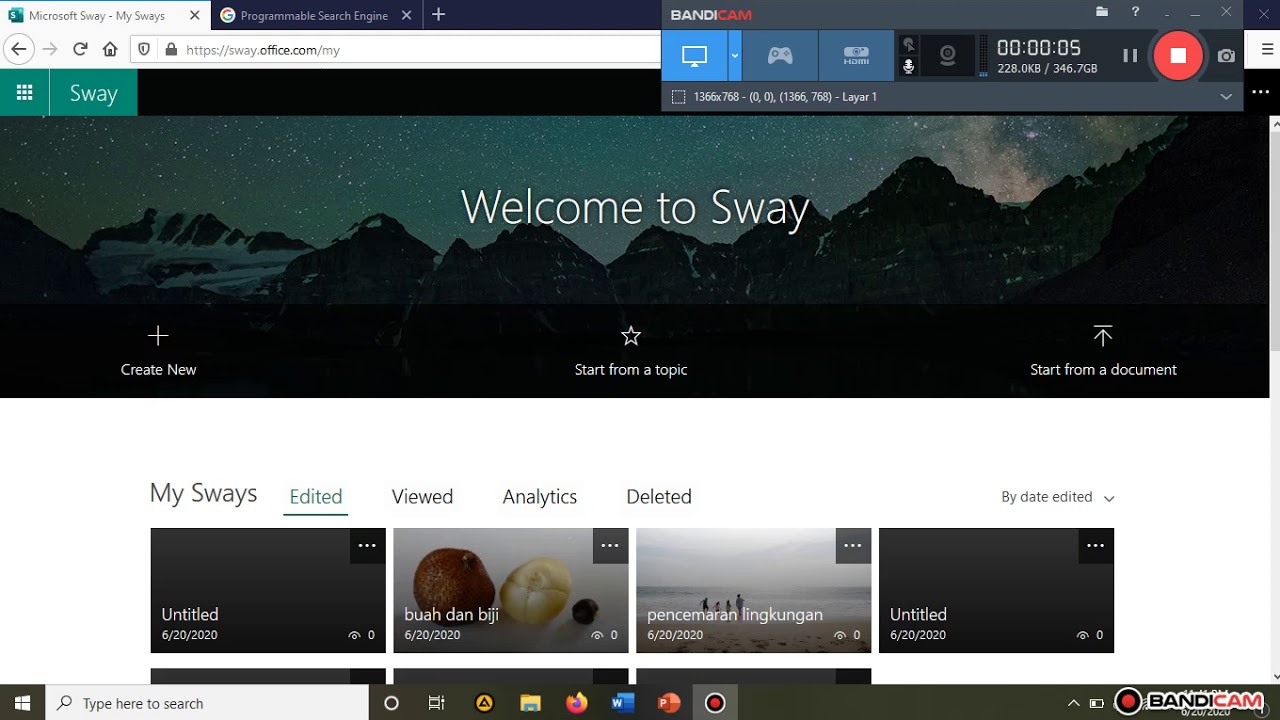The image showcases the user interface of Microsoft Sway, featured at the top of the screen in a gray box labeled "Microsoft Sway" along with the options "My Sways." Nearby, there's a small green box with an 'X' icon, and a green line runs above this section. Navigation icons include a circle with a left arrow, a right arrow, and a return arrow, alongside a house icon. At the very top, a black search box is present, including the Google 'G' icon in its characteristic red, yellow, blue, and green colors, accompanied by the label "Bandicam." Below this, another search box appears, joined by three blue boxes and a counter showing "0000" and "05," accompanied by a small white left arrow. A red circle containing a white box is also visible here, along with a smaller white box with white text below the blue boxes.

Centered in the image is a large picture set against a black background, featuring mountainous scenery with visible smoke. A green drop-down box with nine small dots is labeled "Sway," and the text "Welcome to Sway" is prominently displayed in the middle of this picture. At the bottom, options for creating new content are laid out: "Create New" followed by a white line, "Start from a Topic" with a star icon, and "Start from a Document" with an upward arrow and a line above it.

The user interface continues with a white background displaying the text "My Sways," followed by the underlined options "Edited," "Viewed," "Analytic," and "Deleted.” Below these, four pictures are labeled “United,” “Bush, Dan, BG and Pence,” “Pence, Moran, Ling, Coonga,” and “Untitled.” The right side features a light blue sidebar.

At the bottom of the screen, a small black box with a window and a gray search box is visible. Along the bottom edge, typical icons rest on a black background, including a white box and a white circle with the red text "Bandicam."